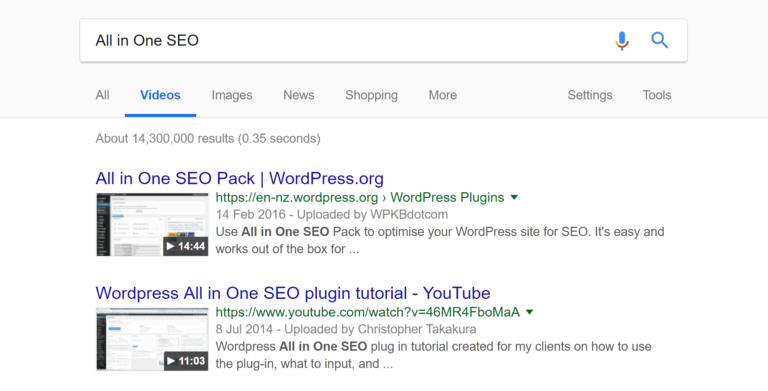A detailed and improved caption for the described image:

"The image features a light gray header at the top of the screen, containing a white rectangle with the text 'All in One SEO' on the left and icons for a microphone and a magnifying glass on the right. Below this header is a navigation bar with 'All' highlighted, followed by 'Videos' in blue and underlined, and then options for 'Images,' 'News,' 'Shopping,' 'More,' 'Settings,' and 'Tools' in gray.

Directly beneath the navigation bar, the search results summary indicates approximately 14,300,000 results found in 0.35 seconds. The first search result is a link in blue text that reads 'All in One SEO Pack - wordpress.org,' with the URL displayed in green beneath it. Additional descriptive text is provided in gray.

To the left of this result is a thumbnail image, resembling a screenshot. Below this, a black rectangle with a pointing arrow icon and the text '14:44' denotes the duration of a video. Below the thumbnail, in blue text, it says 'WordPress All in One SEO Plugin Tutorial - YouTube.' Another similar thumbnail is positioned to the right but features a different duration, which is too small to read clearly. To the right of this second thumbnail, there is another URL in green and additional text in black."

This cleaned-up and detailed caption provides a clearer and more organized description of the visual elements present in the image.